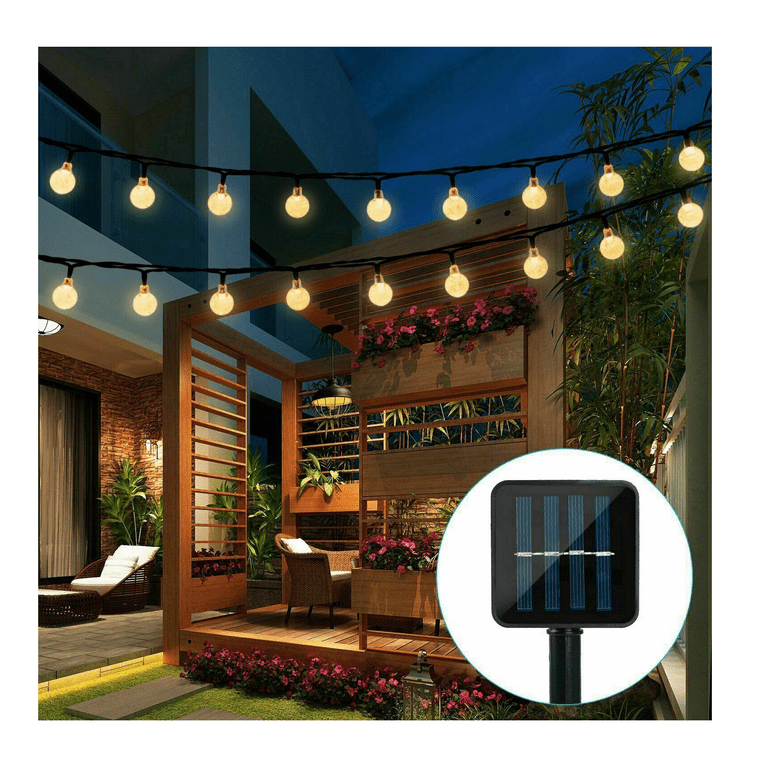This vibrant photograph captures a meticulously designed outdoor seating area set within a landscaped yard, close to a modern-looking house illuminated against the night sky. The primary focus of the image is a wooden-framed, louvered patio structure adorned with built-in planters overflowing with colorful flowers, creating a lush, inviting ambiance. Strung above this intimate space are two sets of bistro lights, casting a warm glow over the wicker chairs equipped with white cushions, enhancing the evening's serene yet lively atmosphere. The seating area features a wooden platform, bordered by additional planters filled with pink flowers, further enriching the scene with their vivid hues. To the left side of the structure, another patio space appears, furnished similarly with wicker chairs, white cushions, and an abundance of plants. A significant element in the foreground is a white circle showcasing a black plastic solar light with four blue solar cells inside, pointing towards an underlying advertisement theme, subtly integrated into this picturesque setting.